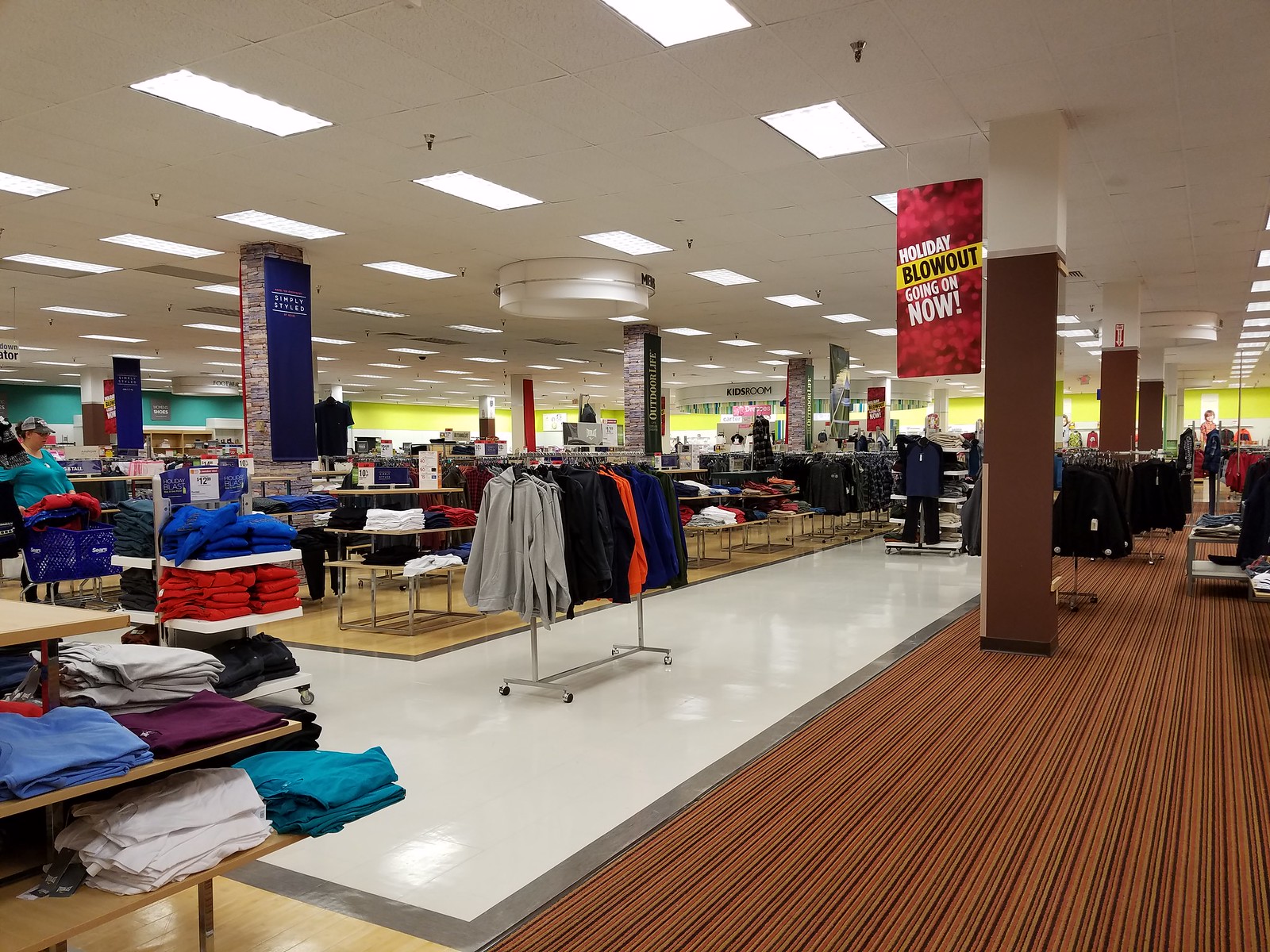The photograph is taken inside a retail store, clearly showcasing the vibrant atmosphere of its clothing section. To the left, a woman is seen pushing a blue plastic shopping cart, distinctive in its bright hue, which matches the store's array of blue carts. In her cart, she has placed a red sweatshirt, adding a contrasting pop of color. The woman herself is dressed casually in a turquoise long-sleeve shirt and a ball cap, her hair pulled back into a ponytail. Surrounding her are numerous clothing racks adorned with a variety of winter outfits, including long-sleeve shirts in shades of gray, black, orange, and blue. Above, the ceiling is covered with white tiles interspersed with fluorescent lights, providing ample illumination to the scene. A prominent sign hangs from the ceiling, reading "Holiday Blowout Going On Now," advertising an ongoing sale. The carpet beneath is a brown striped design, completing the warm and inviting ambiance of the store.